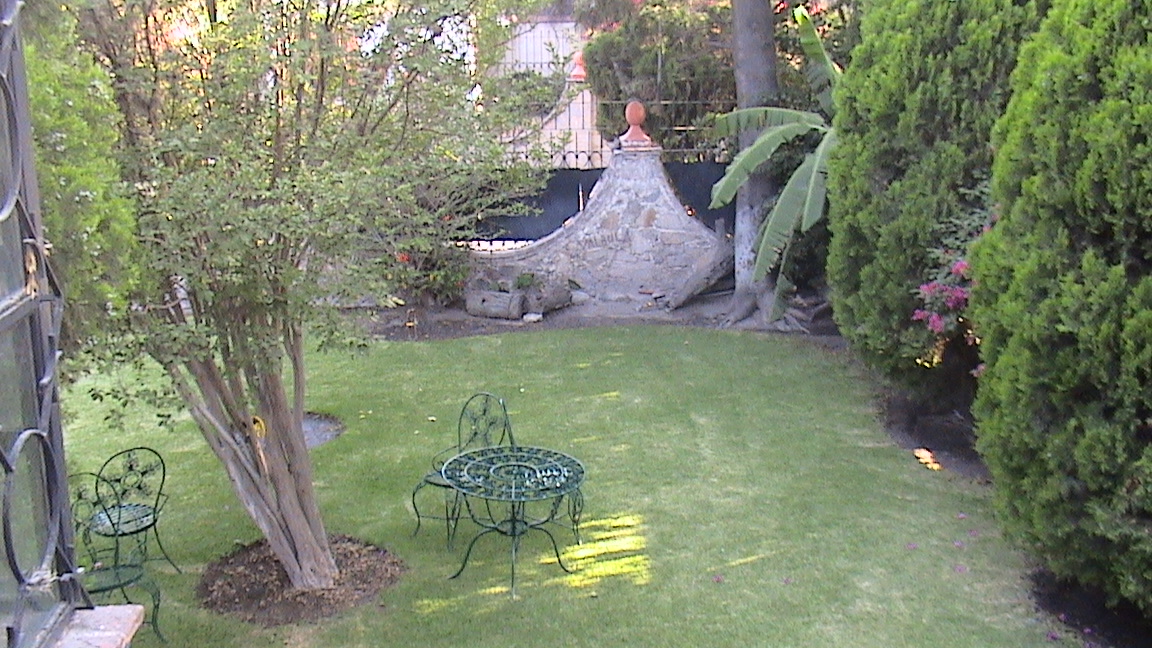This image captures a well-maintained backyard scene, likely taken by a surveillance camera. The short, green grass covers the ground evenly. Dominating the right side of the frame are tall, bush-like plants or possibly small trees, adorned with red and pink leaves. Prominently placed in the center is a green metal table accompanied by a single green chair. To the left of this table stands another tree with sparse foliage and numerous brown trunks, flanked by another green chair. In the backdrop, there's an intriguing gray cement structure topped with a red cement dome-like shape, and a thicker tree trunk to its right. Further to the left, more smaller trees and plants are visible, creating a lush background. In the lower left corner of the image, part of a window with a black metal frame and glass can be seen. Additionally, there are green wire chairs situated in the lower left, adjacent to the solitary tree on that side. The whole scene is bordered at the back by a fence, completing this serene backyard view.